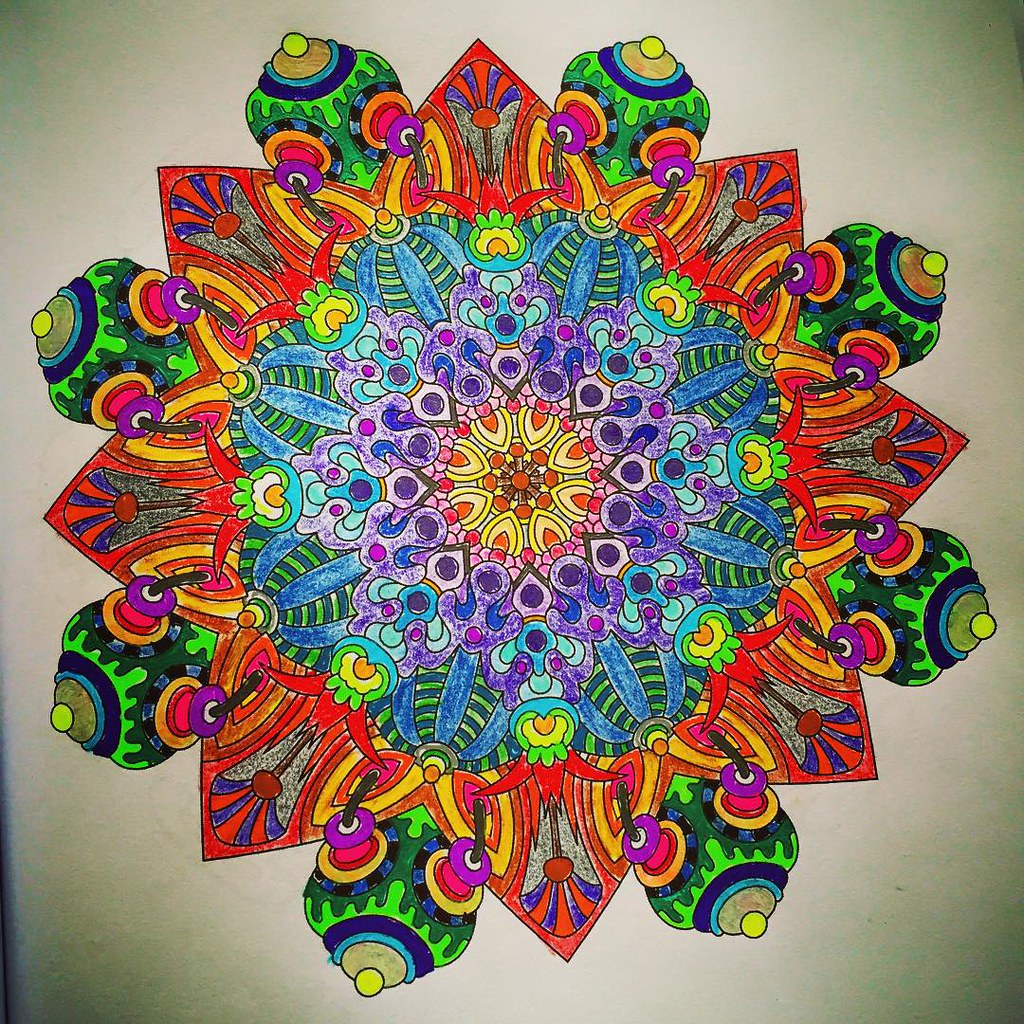This photograph captures a vibrant, meticulously-drawn mandala design on a sheet of white paper, taken from a top-down perspective. The mandala features a stunning kaleidoscope of colors and intricate patterns, creating a symmetrical and repetitive visual effect. The background gradient of the paper shifts from dark, swampy green corners to a light tan center, enhancing the contrast of the design. The center of the mandala begins with a brown core, bordered by medium red, yellow, pink, and various shades of purple and blue. Surrounding these central colors are layers of intricate designs in green, orange, and gold, including petal-like shapes and urn-like figures with green bases and gold lids adorned with blue stripes and yellow tops. The outer edges of the mandala prominently feature orange petals with multicolored interiors, enveloped by vivid hues of green and purple. The entire piece is outlined with a thin black pen and filled in with crayons or colored pencils, resulting in a strikingly colorful and harmonious composition.